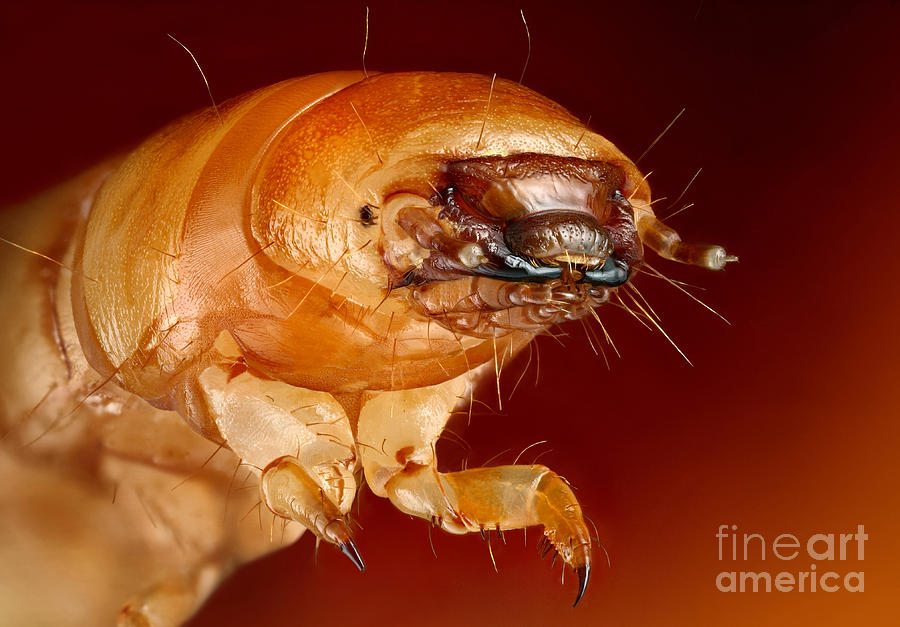This is a detailed, close-up photograph of an insect, labeled "Fine Art America" in lowercase letters positioned in the bottom right-hand corner. The background features varying shades of brown, dark orange, and maroon, contrasting with the insect's distinctive coloration. The insect's body, primarily brown with touches of orange and yellow, is reared up, showcasing the upper portion with two long, tentacle-like appendages at the front, each ending in sharp claws.

The insect is intriguingly detailed, with small, fine hairs adorning its body and face. It has two large, black pinchers near its mouth that resemble fangs, adding to its menacing appearance. Black, beady eyes seem to peer out from its face, enhancing its unappealing and potentially threatening demeanor. The insect's overall appearance is marked by sporadic hairs and needle-like structures, giving the impression that it could sting or bite.